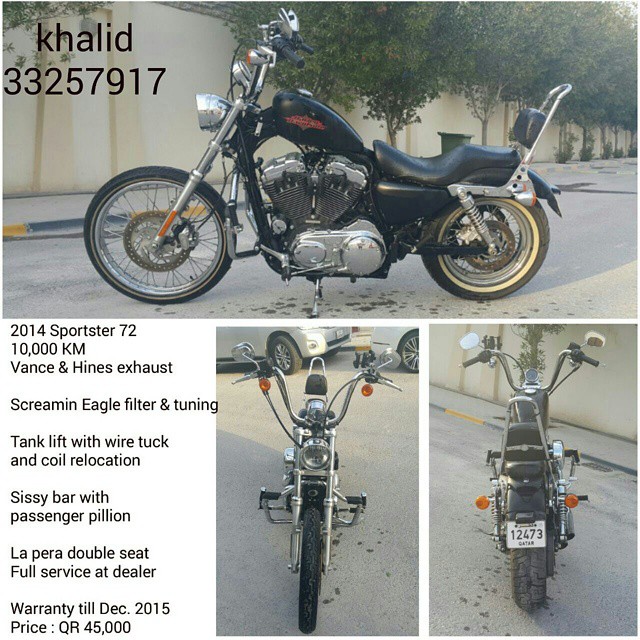The image is an advertisement for a motorcycle, possibly a vintage model, likely posted for sale. At the top of the ad is a horizontal photograph displaying a side view of the motorcycle, with the name and phone number "Khalid 33257917" overlapping in the top-left corner. Below, the ad is divided into three columns: the middle and right columns each contain a vertical photograph of the motorcycle from different angles—one from the front and one from the back. The far left column is a text box detailing the motorcycle's specifics: "2014 Sportster 72, 10,000 kilometers, Vance & Heinz exhaust, Screamin' Eagle filter and tuning, tank lift with wire tuck and coil relocation, sissy bar with passenger pillion, La Pera double seat, full service at dealer, warranty till December 2015, price QR 45,000." The photo on the right also features a license plate that reads "12473 Qatar."